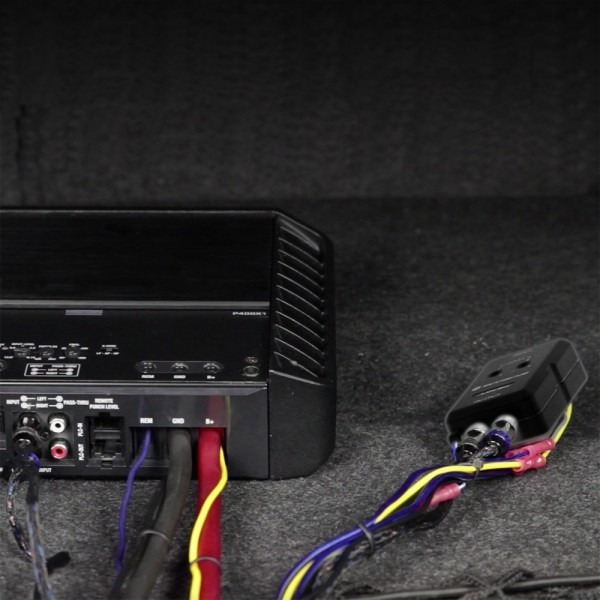In this image, a close-up shows a black electronic device, possibly a receiver, ham radio, or an old VCR/DVD player, placed against a backdrop that resembles a gray or black felt-like material, typical of an audio cabinet or car trunk interior. On the front left of the device, there are visible yellow and red connectors that are unplugged, with another cable emerging to the left of these connectors. Moving to the right, various ports are visible, including what looks like an Ethernet port. Emerging from the back of the box are multiple cords: a purple wire, a larger black wire, and a red wire intertwined with a yellow wire. These wires exit the frame but then reappear alongside additional connectors including a small black box about the size of a palm, to the side. The diverse array of wires and cables connected to this black box device, along with numerous buttons and labels for different inputs and outputs, adds to the intricate detail of the scene, illuminated by light that suggests an open trunk setting where the image is captured.